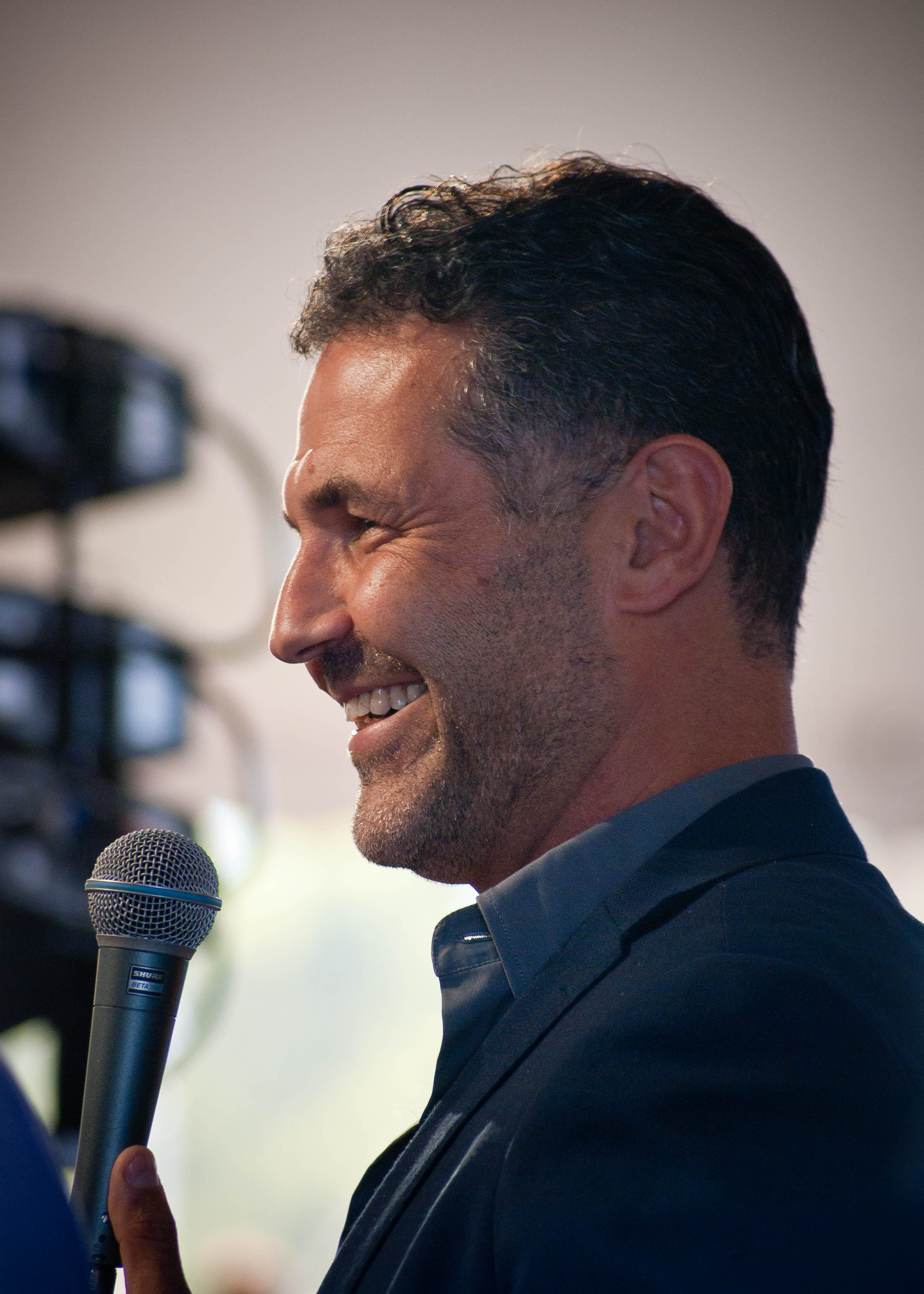The photograph features a middle-aged, white man, approximately in his 40s, with short dark brown hair accented by gray at the temples. He has light stubble on his beard and mustache area. The man is smiling broadly, visibly squinting due to his smile, and is captured in a vertically aligned rectangular frame, showing the left side of his face and shoulder area. He wears a dark blue blazer over a gray button-down shirt. The man is holding a microphone in his left hand, with only his thumb visible on the dark gray base that has a silver top and a blue line across it. Behind him, the background is very blurry, composed of mixed tan, gray, and white hues, with some large black objects—likely lighting equipment or cameras—visible off to the left.